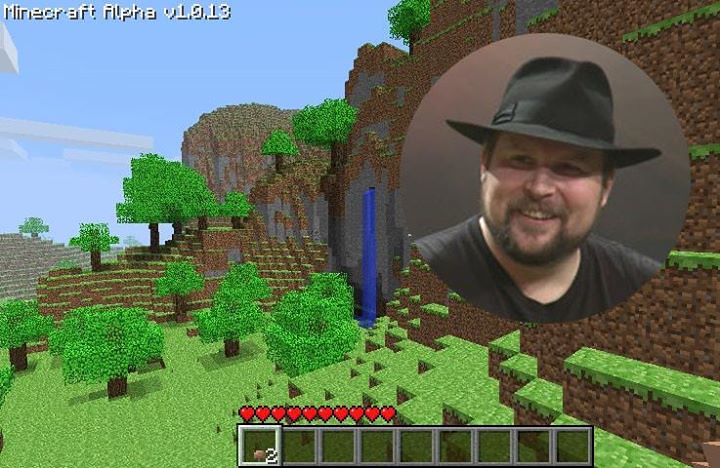A screenshot from Minecraft Alpha v1.0.13 features an overlay of a photograph of a man on the right-hand side. The man is wearing a black top hat adorned with a satin ribbon around the brim, and he has fair skin with a closely cropped mustache and beard. He is smiling, revealing his upper teeth, and is dressed in a dark gray crew-neck sweatshirt. This photograph is superimposed over the Minecraft gameplay.

In the game interface at the bottom, there are nine squares in a row. The first square from the left contains the number "2", while the remaining squares show the game's green background. Above these squares, there are ten red hearts, starting from the left. The terrain in the screenshot is primarily green, interspersed with small brown triangles, and features brown tree trunks with green foliage. A tall, narrow, medium-blue cylinder stands upright in the middle of the screen. In the background, there is a wall composed of mostly brown with patches of green, set against a backdrop of rocks and boulders.